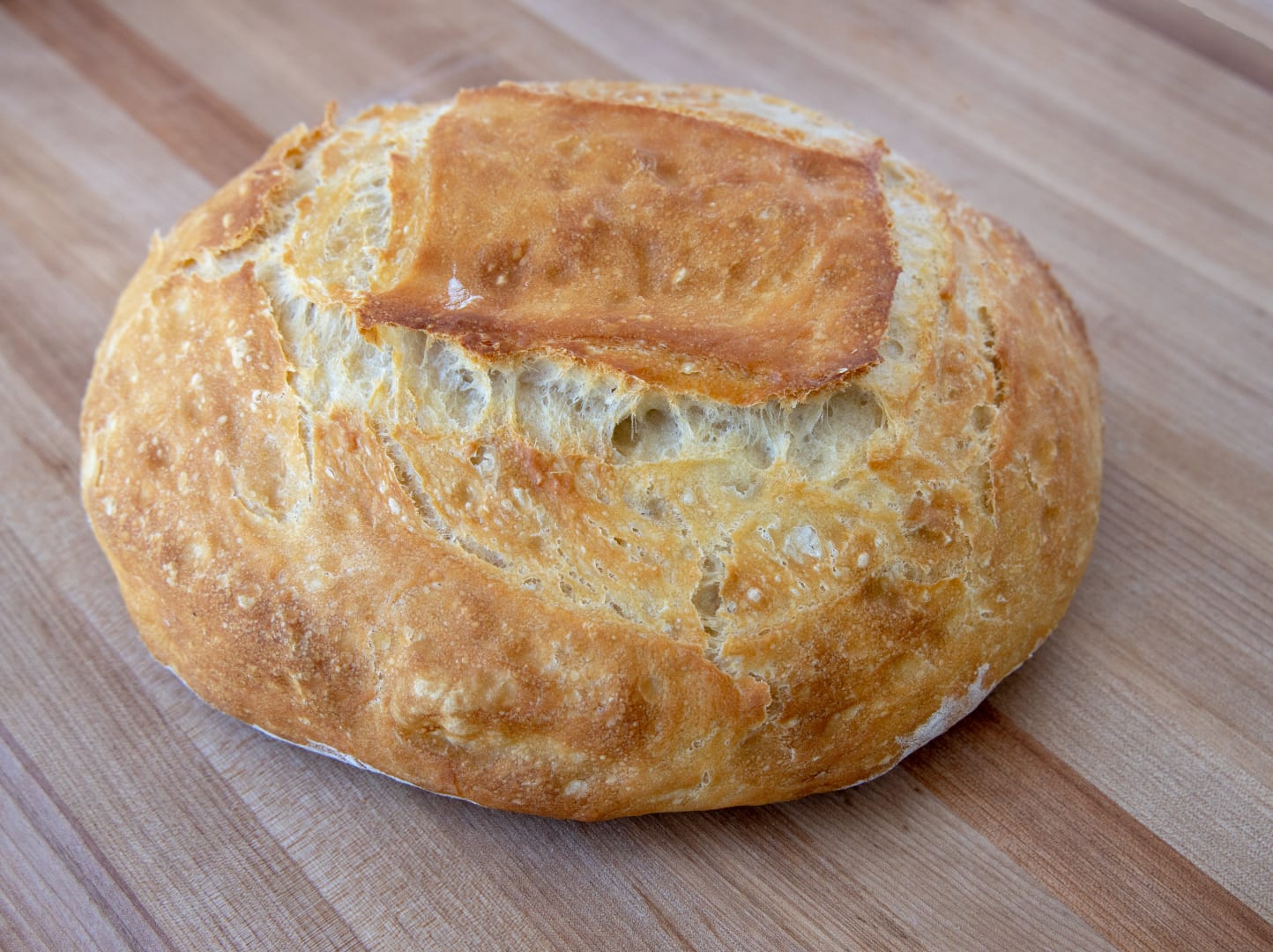This image features a close-up of a large, freshly baked, round loaf of bread resting on a clean, light brown wooden table. The bread is thoroughly browned on the outside, indicating it is well-baked. The top showcases a darker, crispy rectangular spot, with similar crispy and dark areas extending down the sides. The tantalizingly crackly crust reveals hints of the soft, white, fluffy interior through its flaky cracks. A slight dusting of white powder, possibly sugar, can be seen at the bottom of the loaf, adding to its rustic homemade charm. The enticing appearance of this freshly baked bread is enough to make anyone hungry.